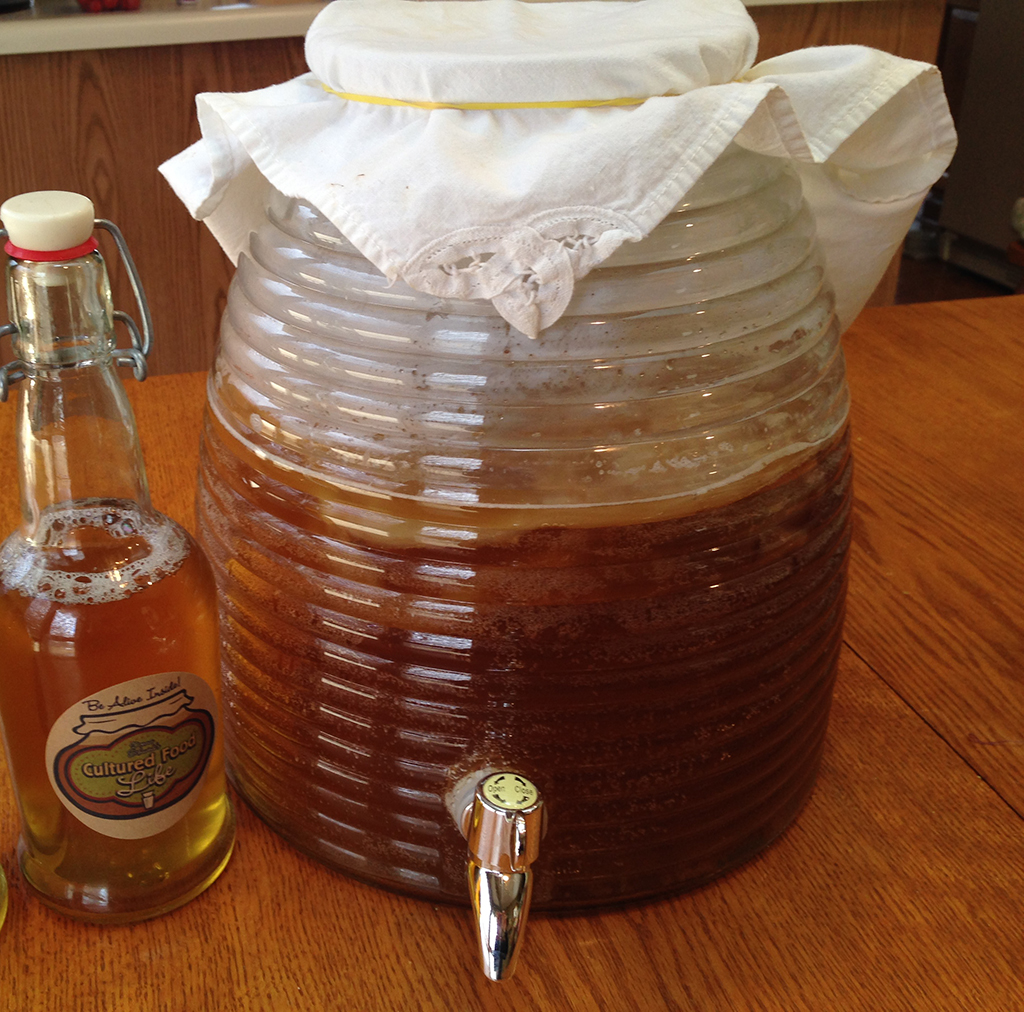The image depicts a drink dispenser and a bottle placed on a wooden table, specifically an oak tabletop. The clear, textured glass beverage dispenser holds a brown, tea-colored liquid, approximately half full. It is fitted with a slightly left-positioned silver spigot, adorned with directional stickers for operation. The dispenser is topped with a light brown cloth, like a napkin, handkerchief, or doily with a laced edge, secured by a rubber band. To its left stands a bottle containing a similarly colored liquid, but lighter, potentially due to lighting. This bottle is semi-filled and exhibits bubbles at the top, suggesting fermentation. It features a label that reads "cultured food life" in yellow and white text beneath cursive writing that is partially illegible. The bottle’s design, with latches, indicates it can release pressure to prevent breaking, common in fermented drinks such as root beer or other probiotics. In the background, another wooden counter with a white top and some indistinct items, possibly red or orange, can be seen.